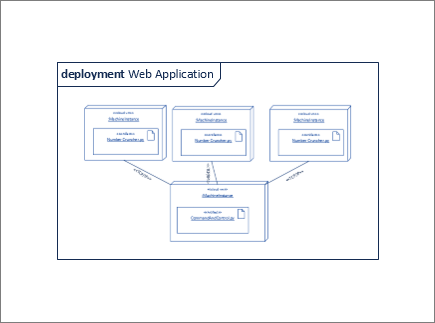This image is a detailed diagram set within a layered black-framed rectangle structure. At the center, an inner white rectangle showcases a clearly labeled infographic. At the top of this infographic, there's an oval-shaped text bubble reading "Deployment Web Application," with "Deployment" in bold text and "Web Application" capitalized. Beneath the text bubble, the diagram features three horizontally aligned, three-dimensional smaller rectangles outlined in blue. These rectangles are predominantly white with blue text, though the text is not legible. Connecting to each of these smaller rectangles are black lines that lead down to a slightly larger, similarly white and blue, three-dimensional rectangle at the bottom. The overall layout suggests a hierarchical or flowchart structure, indicating that the three upper elements are integrally connected to the lower element.